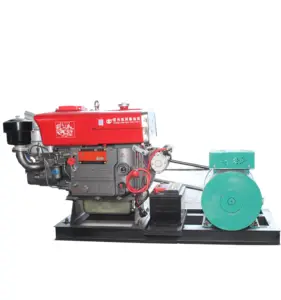The photograph depicts an intricate power generation setup mounted on a black metal frame constructed from welded I-beams. The central component is a compact engine, primarily silver with a prominent red feature on top, believed to be a fuel tank with a nozzle. Attached to the engine is a black air filter. Adjacent to the engine is an aqua-colored, possibly metallic generator connected via a pulley system with a drive belt. Positioned between the engine and the generator is a 12-volt automotive battery, with cables running from it, likely integral to the system's operation. The entire assembly, set against a white background, highlights a foreign script on the red tank, suggesting Asian origin, possibly Chinese. Wires are visible, contributing to the complexity of the machinery, with the setup clearly designed for power generation purposes.